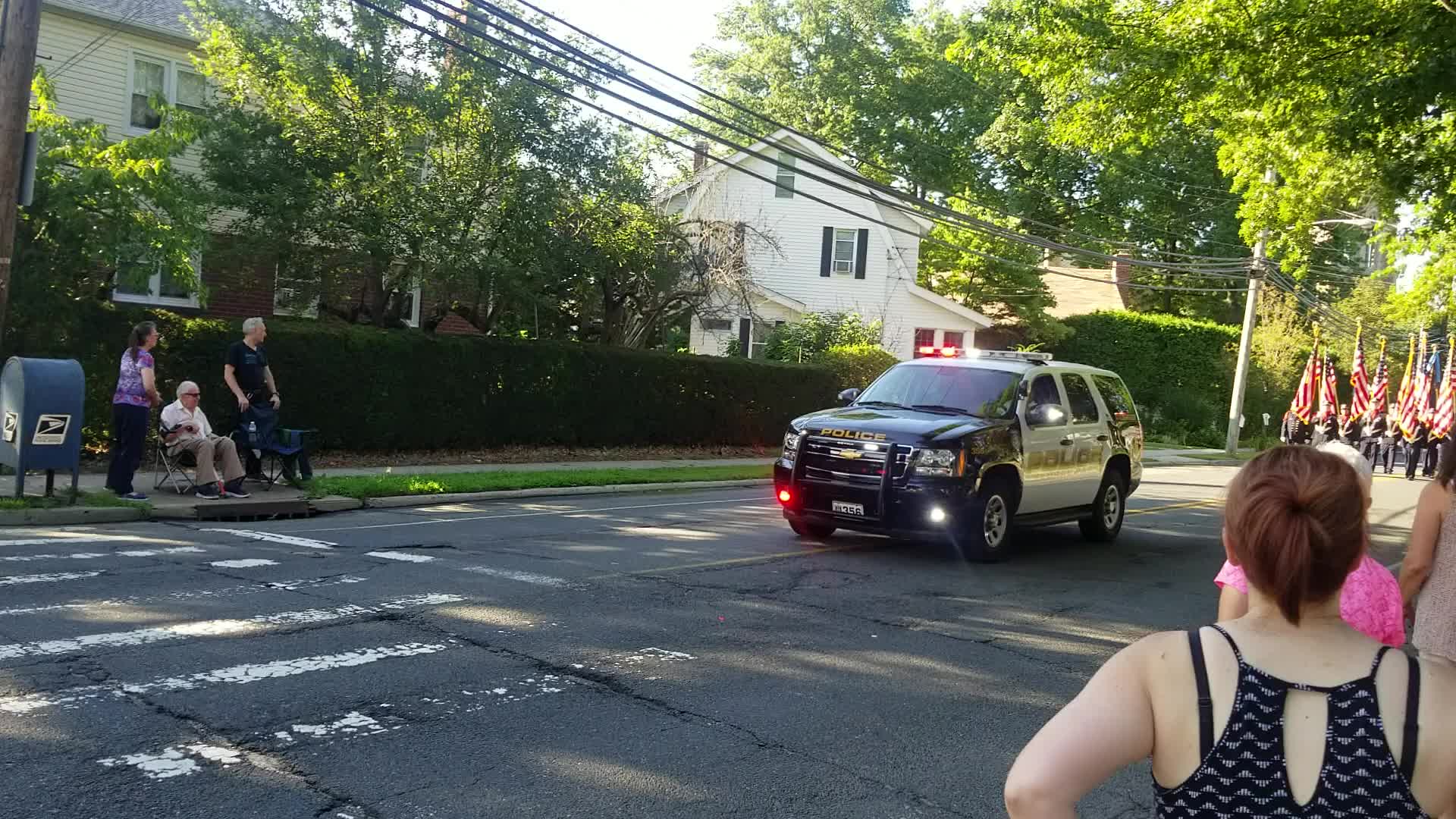The image captures the beginning of a solemn yet respectful procession, likely a funeral parade, taking place in a residential neighborhood. The scene is anchored by a police SUV with its emergency lights on, possibly a Chevy Tahoe, leading the way. On both sides of the street, people gather to observe the procession. On the left side, a mailbox stands beside a woman wearing a purple shirt, near an older gentleman seated on a chair, and another man in a black shirt standing nearby. Across the street, more observers, including a man sitting down, watch attentively. The background is lined with well-kept bushes and trees, typical of a suburban setting. Behind the police vehicle, uniformed individuals march, each holding an American flag, adding to the ceremonial atmosphere. This convergence of community members, flags, and law enforcement indicates a respectful tribute, reinforcing the likelihood of a funeral procession.